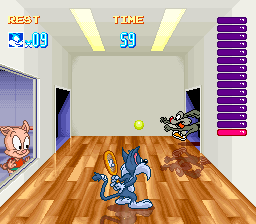This image is a detailed screenshot from a video game. At the top of the screen, there are two sections, each with a large label: "REST" on the left and "TIME" on the right. Below these labels, numeric values are displayed in blue with "09" beneath "REST" and "59" beneath "TIME." The central focus of the image features a character resembling Wile E. Coyote, who is holding a tennis racket while standing on a wooden plank floor. Above this character, a greenish-yellow tennis ball is in mid-air.

To the right of Wile E. Coyote's character, another animal character is emerging from a room. On the left side of the screen, there is another room opening that is highlighted in purple. Through a window near this purple opening, another animal character, resembling a pig with very wide, oval eyes, is peering inside.

The right side of the room is adorned with a vertical column of rectangular items, mostly purple, with the last one in the column being red. The room itself is illuminated by fluorescent lights, and the walls are painted white, giving a sterile, bright environment.